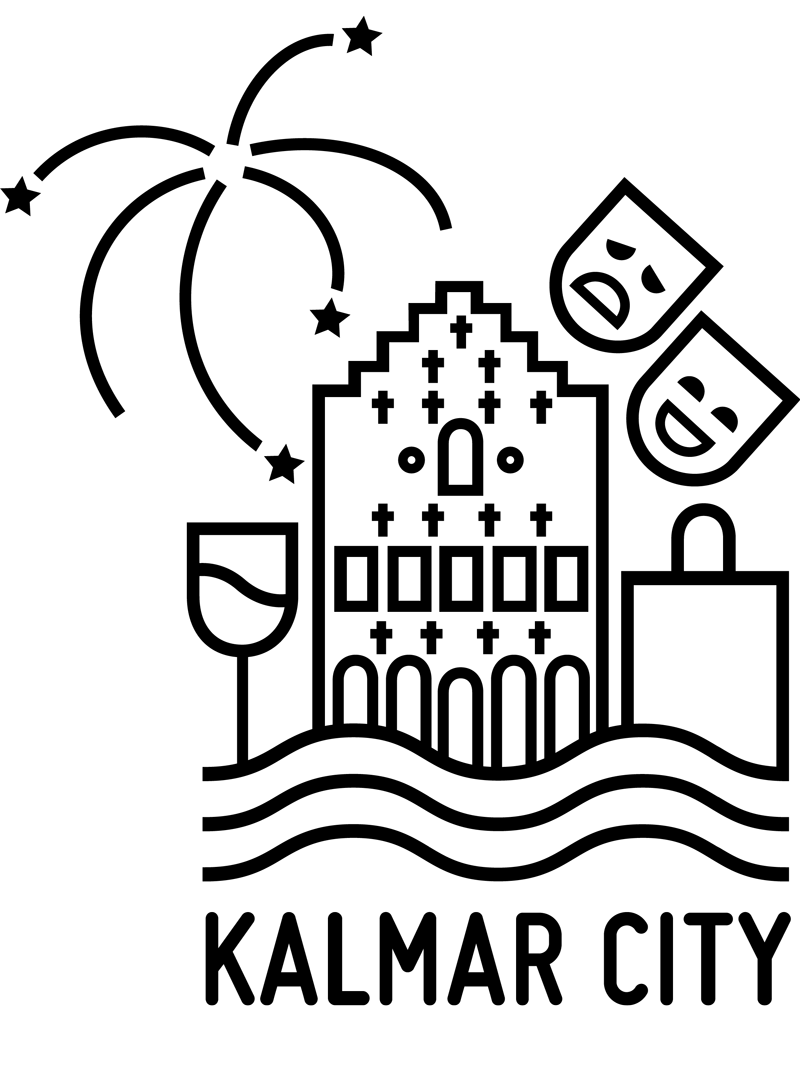This black and white computer-generated graphic, almost like a logo, depicts a large cathedral-like building at the center, featuring numerous arched doorways, various windows, and several crosses throughout its structure, including a prominent arched window at the building's peak. To the left of the building is a goblet resembling a wine glass filled with fluid, while to the right stands a depiction of a shopping bag. Above the building, to the right, are the theater tragedy and comedy masks, symbolizing entertainment, with the sad face on the left and the happy face on the right. To the top left, there are fireworks illustrated with lines ending in stars. Beneath the building, goblet, and shopping bag are three wavy lines, possibly indicating proximity to water or a riverside. The entire design is set against a white background with all elements rendered in black. Below the image, the text reads "Kalmar City".